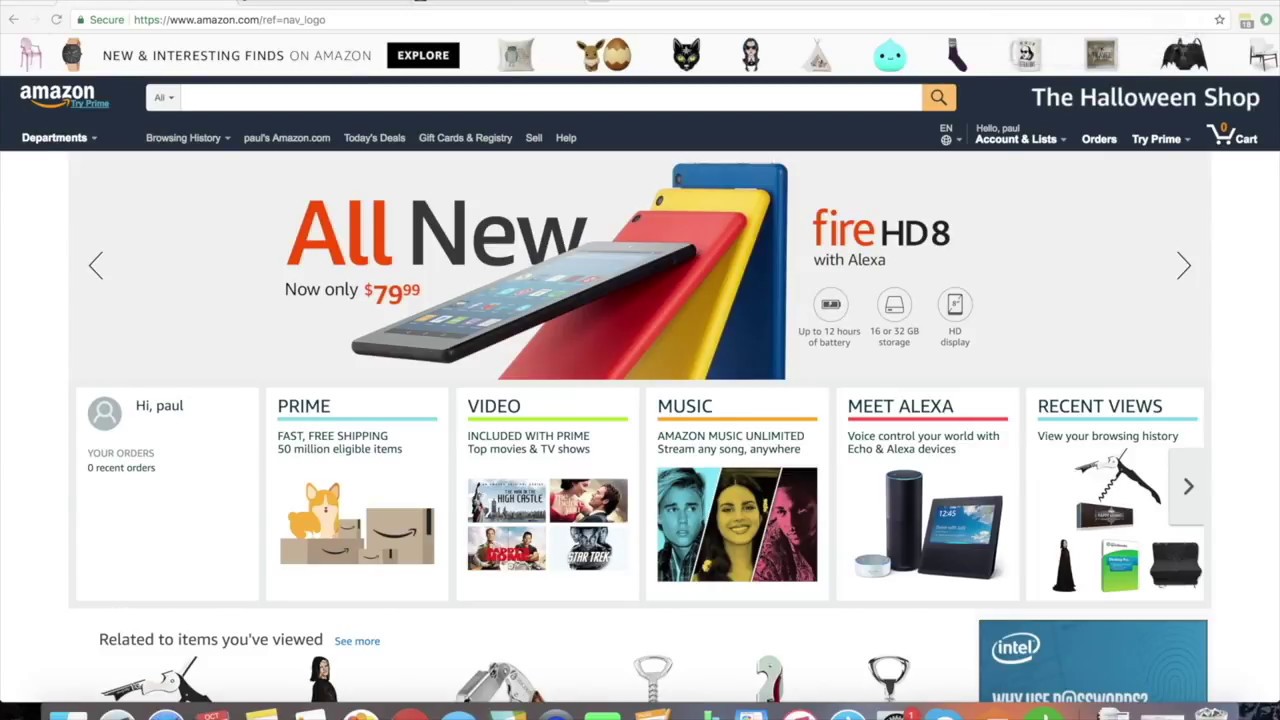A comprehensive screenshot of an Amazon store webpage displayed on a PC screen showcases a multitude of elements, providing an intricate look into various features and products available. 

At the top of the page, a navigational bar outlines various categories, beginning with images of a chair and a wristwatch labelled "New and Interesting Finds on Amazon." An 'Explore' button is prominently displayed next to these items, inviting users to browse further. Following this, there are small icons of a pillow, a horse, an egg, a black cat face mask, another chair (which appears to be a gamer’s chair), a white bag, a blue bird face, socks, a pillow, a picture frame, and an indiscernible last icon.

Beneath the navigational bar, a promotional banner captures the viewer’s attention with an advertisement for "Amazon All-in-One" available for "now only $79.99." Featured in this section is the Fire HD 8 with Alexa, appearing similar to a tablet rather than a phone. It showcases various color options, including black, red, yellow, and blue.

To the right of this banner, a personalized greeting reads, "Hi Paul, your store's 9 recent orders," indicating a customized user experience. Below this is a row of categories: "Prime," "Video," "Music," "Meet Alexa," and "Recent Views," offering quick access to Amazon's services and previously viewed items.

The detailed screenshot offers a visually rich representation of the Amazon online store, demonstrating its wide array of products and features designed to engage and assist customers.